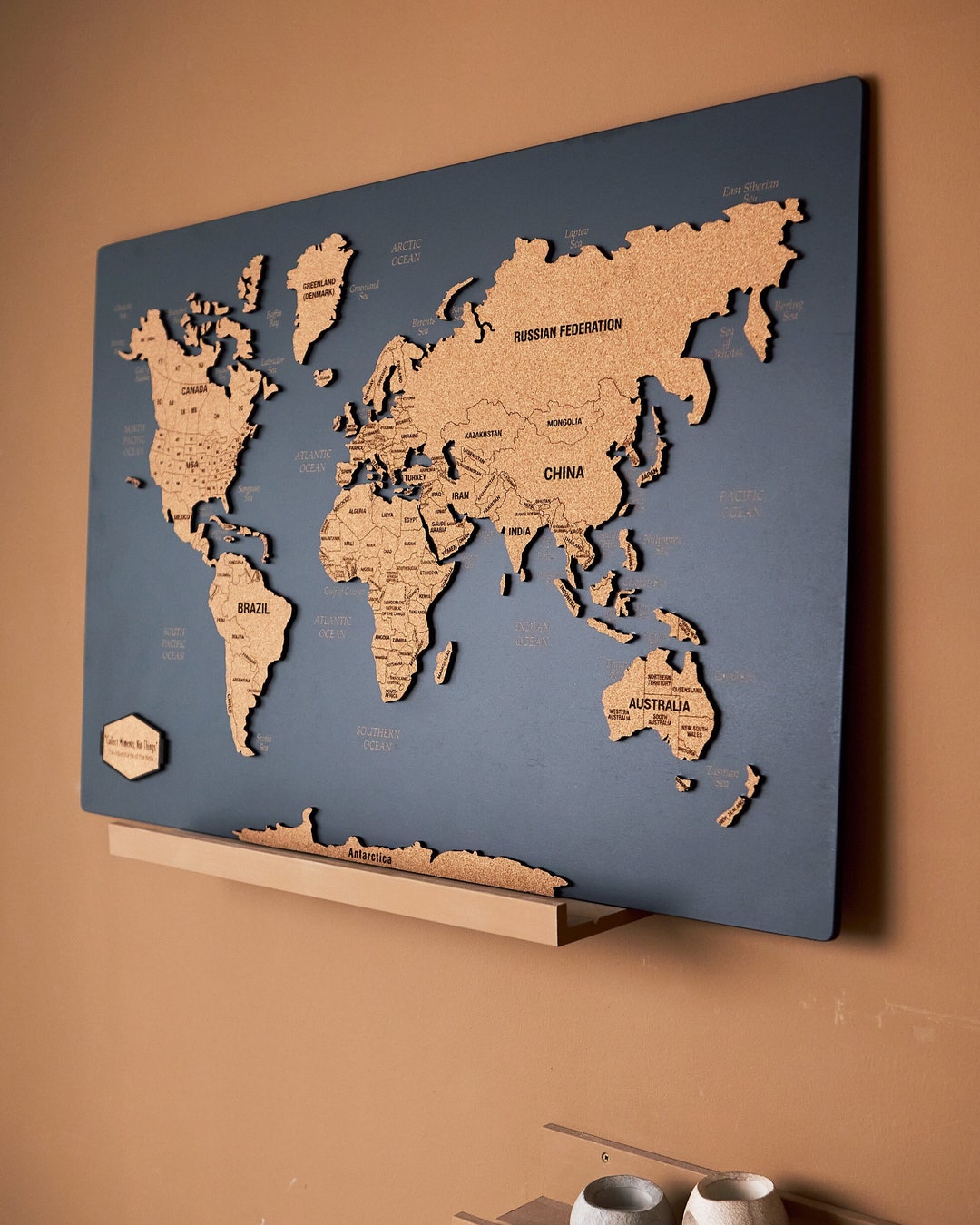This detailed image depicts a visually striking map displayed on a camel brown wall. The map itself is set on a dark background, which could be black or dark blue, and it rests on a small shelf or platform. The raised map pieces, rendered in a golden camel brown, detailedly illustrate various countries including Brazil, Australia, China, India, the Russian Federation, Canada, the USA, Mexico, and Greenland. The surrounding oceans, such as the Atlantic Ocean, South Pacific Ocean, and the Southern Ocean, are labeled on the dark gray areas of the map. At the very bottom, Antarctica is depicted, alongside the tip of Australia and its island. Below the map, a secondary wooden platform houses circular bowls, possibly made of clay or wood, that could be mistaken for candles or cups.